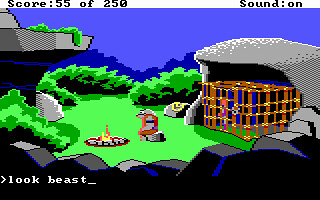This screenshot from a retro-style 2D video game depicts a pixelated outdoor scene set in a grassy clearing amidst mountains with a blue daytime sky. A small rock-surrounded fire pit with pixelated flames occupies the center, where a character is seated on a rock or stump, facing the fire. To the right, there is a stone cave entrance housing a wooden cage constructed with sticks and yellow bands. Surrounding the clearing are low trees and bushes, adding a touch of greenery. The bottom of the image features large rocks framing the scene, while on the far left and the top of the image, white text on a black banner displays “look > beast_” and “score 55 of 250” respectively. The upper right corner confirms the sound status with the text “sound: on.”